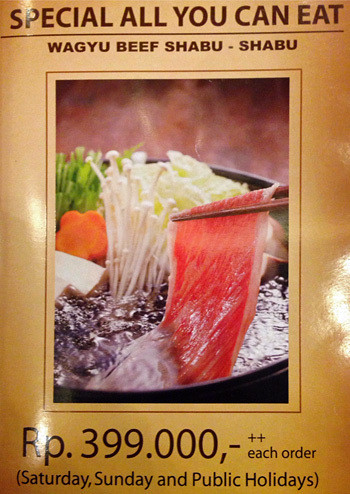The image is a glossy promotional poster with a light beige background and dark brown print, featuring a special offer for an all-you-can-eat Wagyu Beef Shabu Shabu. At the top, "Special All-You-Can-Eat" is prominently displayed in dark text, underlined by a thin horizontal line stretching across the poster. Below this, the text reads "Wagyu Beef Shabu Shabu." Central to the poster is a rectangle outlined with a pinstripe, containing a detailed photograph of a steaming hot pot. In this hot pot are white kinoko mushrooms, thinly sliced red beef, green onions, carrots, and another white vegetable. The photograph captures the richness of the ingredients, with steam visibly rising from the dish. Below the photograph, the price is listed as "RP.399.000," followed by a hyphen and "++ each order." In parentheses, it specifies that this offer is available on "Saturday, Sunday, and public holidays."